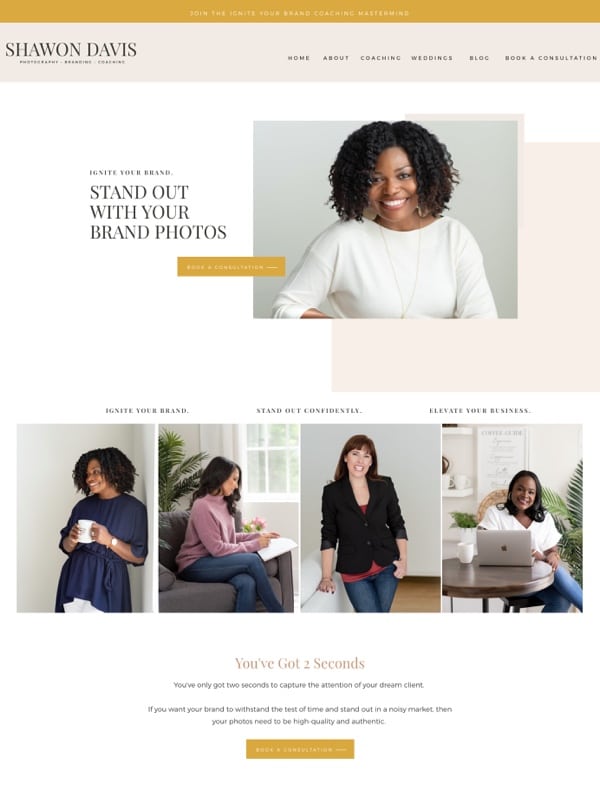The photo showcases Shawan Davis’s website, focusing on her photography and brand coaching services. At the top, a beige bar invites visitors to "Join the Ignite: Ignite Our Brand Coaching Mastermind." Just below the website’s header, a photo of Shawan Davis, an African American woman with curly hair parted down the center, is featured prominently. She is smiling brightly and is adorned with a large gold chain and a white long-sleeved top.

To the right of her name, a menu bar includes the options: Home, About, Coaching, Weddings, Blog, and Book a Consultation. The text is slightly hard to read. To the left, the headline "Ignite Your Brand" is displayed on a white background, accompanied by a subhead that reads, "Stand out with your brand photos," and a call-to-action button overlaying this white section and her picture.

Beneath this are four photographs under the bold heading "Ignite Your Brand." They emphasize the message "Stand out confidently, elevate your business." The first photo shows Shawan Davis leaning against a wall. The second image features a woman, possibly Caucasian or Asian, standing in front of a couch facing forward. The third depicts another Caucasian woman, potentially with red or brown hair. The last image features another African American woman seated at a brown table with a sleek laptop in front of her.

At the bottom, a highlighted text message stresses, "You've only got two seconds to capture the attention of your dream client. If you want your brand to withstand the test of time and stand out in a noisy market, then your photos need to be high quality and authentic." There is a call-to-action text that likely reads, "Book a Consultation," though it is somewhat difficult to decipher.